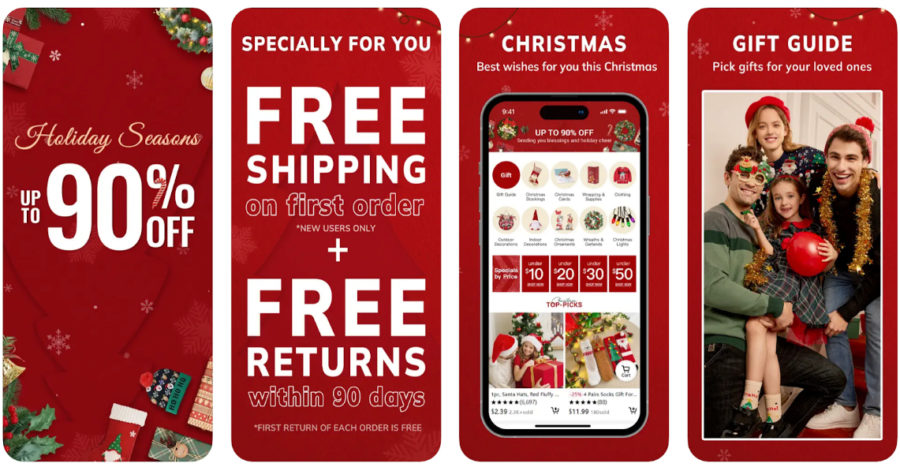The image comprises four vertical, cell phone-shaped rectangles arranged side by side, serving as an advertisement for a store's Christmas sale. Each rectangle features a dark holiday red background.

- The first rectangle on the left is decorated with festive elements such as presents, stockings, hats, and other Christmas-themed items in the corners. At its center, the text announces, "Holiday Seasons - Up to 90% Off."

- The second rectangle also has a red background and features white text that reads, "Especially for you, free shipping on first order." Below that, a plus symbol and additional text state, "+ Free returns within 90 days."

- The third rectangle displays an image of a black and gray cell phone. At the top, it reads, "Christmas, Best Wishes for You This Christmas." The cell phone screen shows a website featuring various Christmas items and their prices, underscoring the theme of the sale.

- The fourth rectangle on the right starts with the text "Gift Guide" in white at the top. A string of Christmas lights adorns the upper right corner of the image. It continues with the message, "Pick gifts for your loved ones." Below, there's a horizontal picture of a family dressed in humorous Christmas hats, wrapped in garland. The family consists of a man, a woman, a teenager, and a young girl sitting on the man's lap, holding a red ball.

The overall design exudes a festive holiday spirit while promoting a significant sale and additional perks for shoppers.